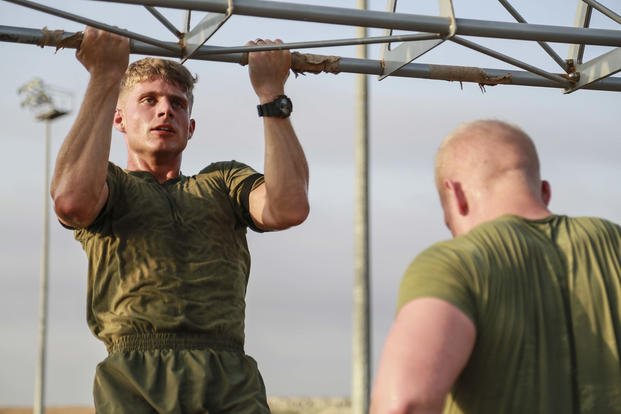The photograph captures a military training scene featuring two men in green fatigue-like t-shirts, possibly shorts, performing exercises. The focal point is a muscular man with closely cropped hair on the sides and a bit more on top, wearing a black watch on his left wrist, who is mid-pull-up on a sturdy, metal girder structure. He is visibly exerting himself, with tense muscles and a determined expression. In front of him stands another man, seen only from the back, similarly attired in a green t-shirt, which is darkened with sweat. This second man, whose hair is trimmed short, appears to be guiding or counting for the man doing the pull-ups. The background features a gray sky with a few light poles or observation posts, adding to the military ambiance of the outdoor training setting.